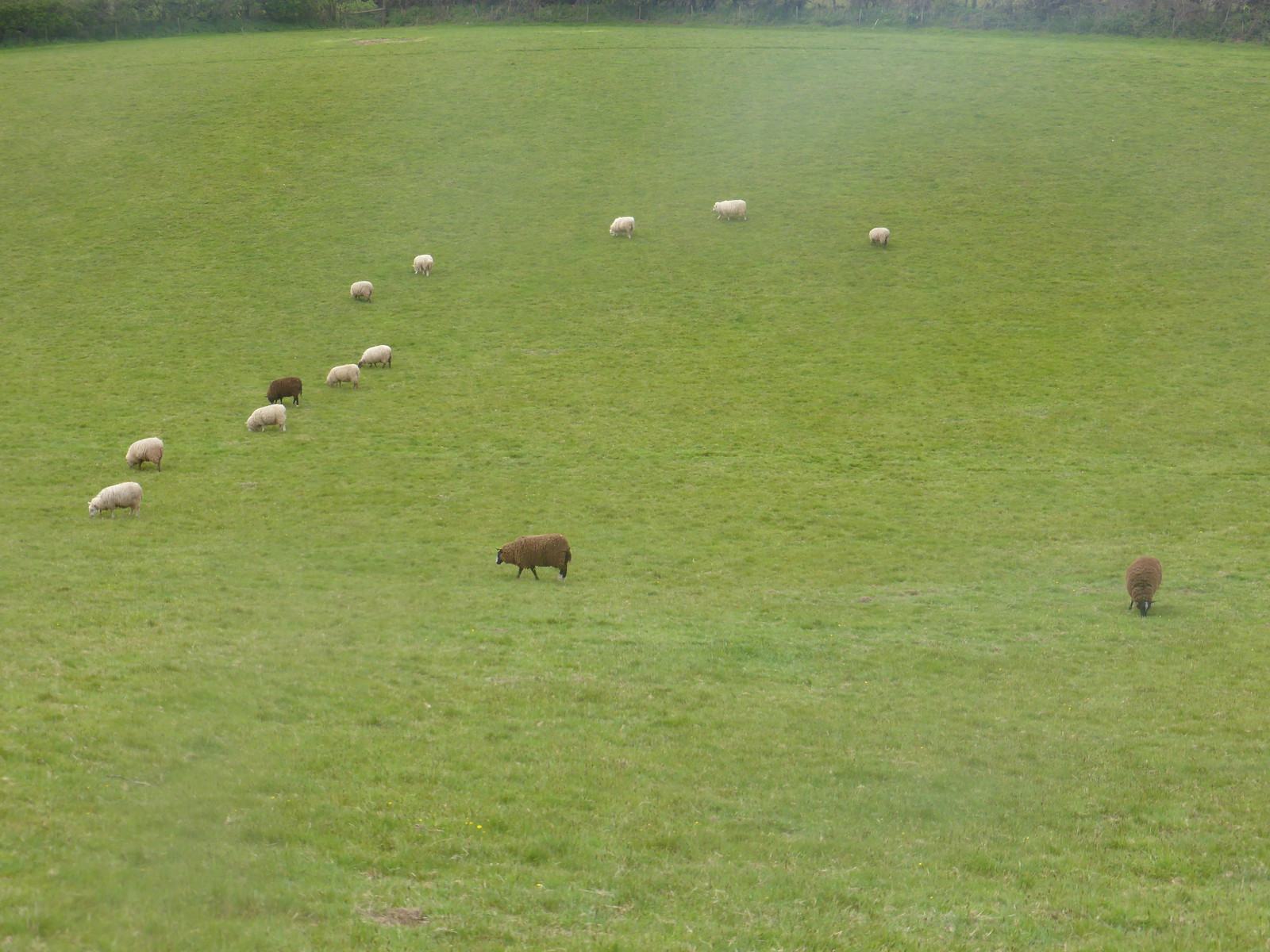The photograph depicts a serene, flat field of vibrant green grass under a sunny sky. Spread across the field are 13 adult sheep, where 10 are white and 3 are brown. Among the white sheep on the left side, there is one brown sheep intermingling. Another brown sheep is centrally placed, grazing alone, while the remaining brown sheep is situated alone on the right. All the sheep appear to be feeding on the grass. In the background, at the very top of the image, a dense strip of darker vegetation suggests the beginning of woods or thicker bushes, creating a subtle contrast to the openness of the field. The day is bright and clear, with no shade present, enhancing the lushness of the grass and the distinct colors of the sheep.